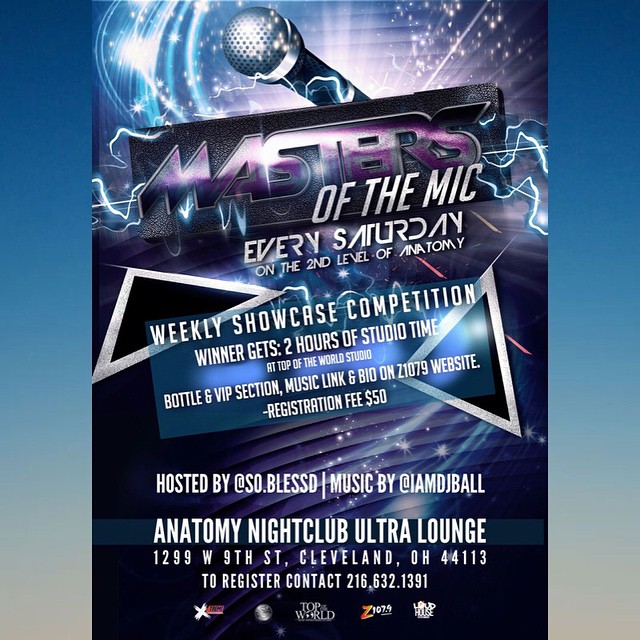The advertisement is for an event at the Anatomy nightclub and ultra lounge, featuring a vibrant design centered on a gripping visual. The background starts with a deep, dark blue that fades into a tan hue near the bottom, setting a dramatic tone. At the very top, blue and purple hues dominate, adorned with bright lines and stars, exuding a vibrant energy. In the center, a powerful image of a microphone with a black handle and a silver top takes prominence, from which a striking bolt of lightning emanates.

Beneath this, a black text box displays the event's title in an eye-catching large purple and black font, declaring "Masters of The Mic." Silver lettering beneath it highlights the timing: "Every Saturday on the second level of Anatomy." A light blue box nestled under this provides further details with white lettering about the "Weekly Showcase Competition."

The poster also lists additional information: "Hosted by @SoBlessed, music by @IMDJBall," and details about the prizes: "Winner gets two hours of studio time at Top of the World Studio, bottle and VIP section." It also provides logistical details including the venue's address, "Anatomy Nightclub Ultra Lounge, 1299 West 9th Street, Cleveland, Ohio 44113," and a registration fee of $50, with contact information for registration at "216.632.1391," directing potential participants to a music link available via a C1079 website.

With a bustling and detailed composition including 3D illustrations and text elements like dark triangles with silver borders, the ad leaves an impression of electrifying anticipation for the event.